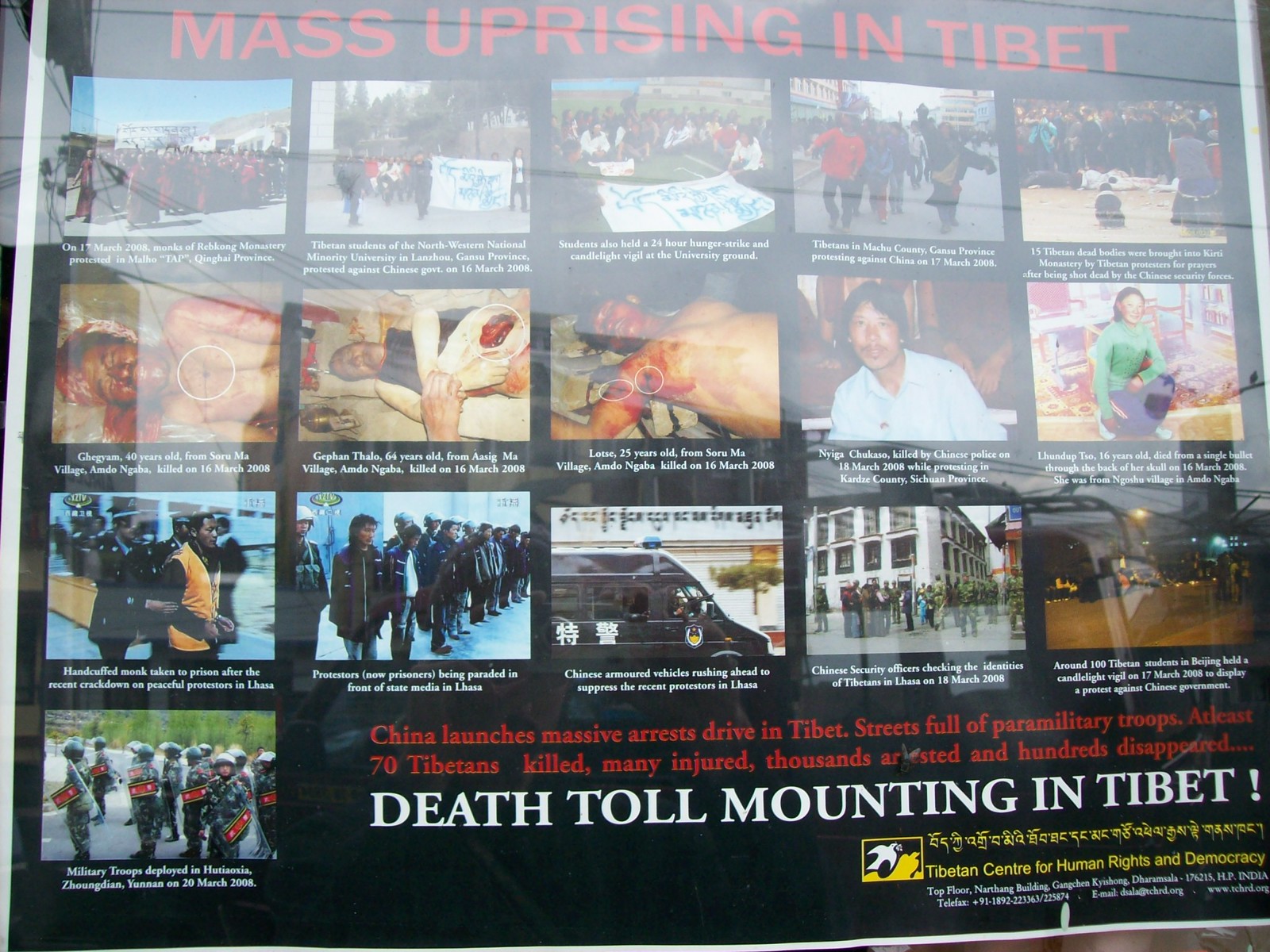The image appears to capture a poignant outdoor scene, as evidenced by reflections hinting at an outdoor background. Dominating the top of the banner, a somber black border frames the stark red text proclaiming, "Mass Uprising in Tibet." The central portion of the banner is a grid featuring twenty disturbing photographs, arranged in five rows and four columns, documenting harrowing events occurring in Tibet.

In the bottom right-hand corner, the red text provides a grim update: "China launches massive arrest drive in Tibet, streets full of paramilitary troops, at least 70 Tibetans killed, many injured, thousands arrested, and 100 disappeared." Amplifying the sense of urgency, another bold message sprawls across the banner in large white letters: "Death Toll Mounting in Tibet."

Beneath this declaration, yellow text presents a message in another language, which is not translated. Following this, in English, it reads: "Tibetan Centre for Human Rights and Democracy." The banner as a whole serves as a stark, visual account of the ongoing crisis, amplifying the cries for awareness and action concerning the human rights situation in Tibet.